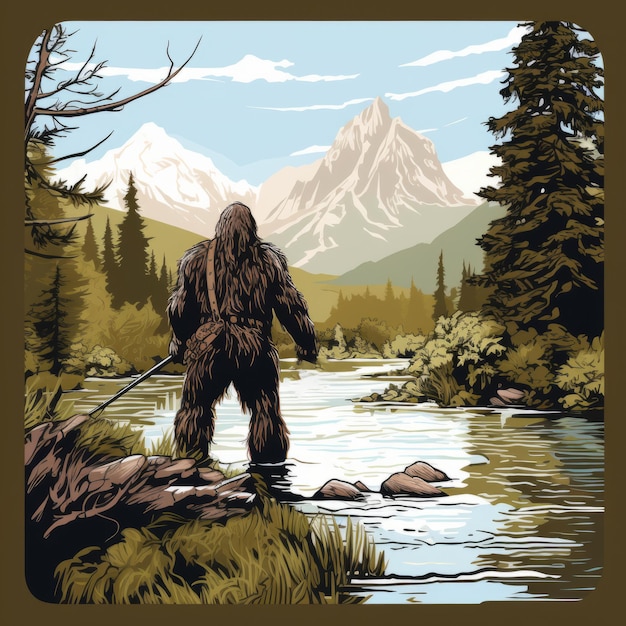The image features a computer-generated graphic depicting a majestic scene where a large, wookie-like creature, reminiscent of Chewbacca from the Star Wars saga, stands with its back to the viewer. This towering figure, which could also be interpreted as a Sasquatch or a brown yeti, is adorned with a small brown satchel slung across its shoulder. The creature is positioned in the middle of a serene creek, which is lined with smooth stones and flanked by lush wilderness. Encompassing the creek are tall, verdant pine trees and a variety of plant life, creating a rich tapestry of nature. In the distance, imposing snow-capped mountains rise against a clear blue sky with fluffy white clouds scattered across. This enchanting landscape evokes a sense of adventure and tranquility, as the creature gazes contemplatively at the distant peaks.